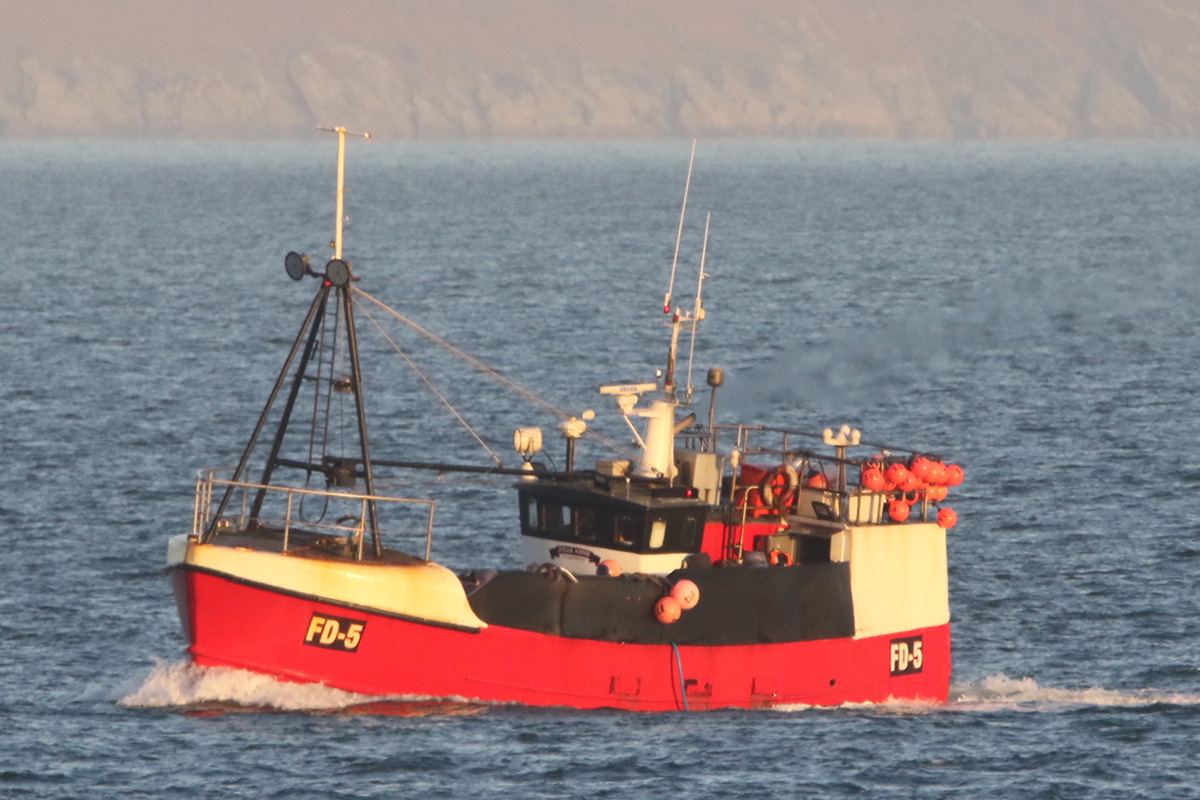A striking image captures a medium-sized sea vessel identified by FD5 inscribed in white text on black rectangular boxes at its front and back. The boat, characterized by its prominent red bottom, and black and white upper structure, cuts through dark blue waters with noticeable waves both at the bow and stern, suggesting it is powered. The vessel is adorned with orange, buoy-like objects, especially toward the back and sides. There are also triangular projections and antenna-like structures rising from its deck. The backdrop is a rugged, gray, mountainous landscape, sprinkled with snow, hinting at cold weather. The scene is distinctly maritime, conveying the vessel's journey through a large, icy body of water.